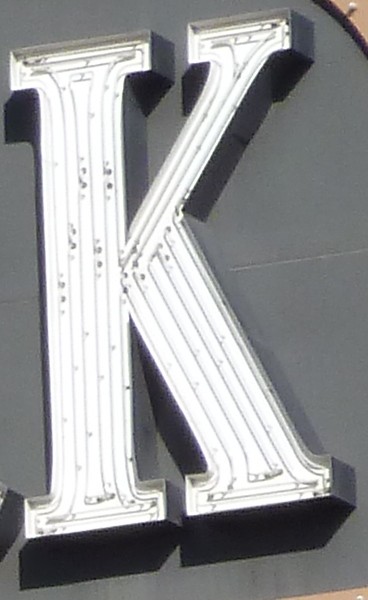This photograph captures the exterior of a building or store featuring an unilluminated neon sign during the daytime. The main focus is a prominently displayed white letter "K," with intricate neon tubes outlined within the letter. Just the edge of an adjacent letter is visible to the left, suggesting the sign consists of more characters. The letter "K" and its neighboring letter are encased in a circular black frame, hinting that the letters belong to a larger, cohesive sign. The composition draws attention to the craftsmanship of the neon tubes and the stark contrast between the white letter and the black framing, all bathed in natural daylight.